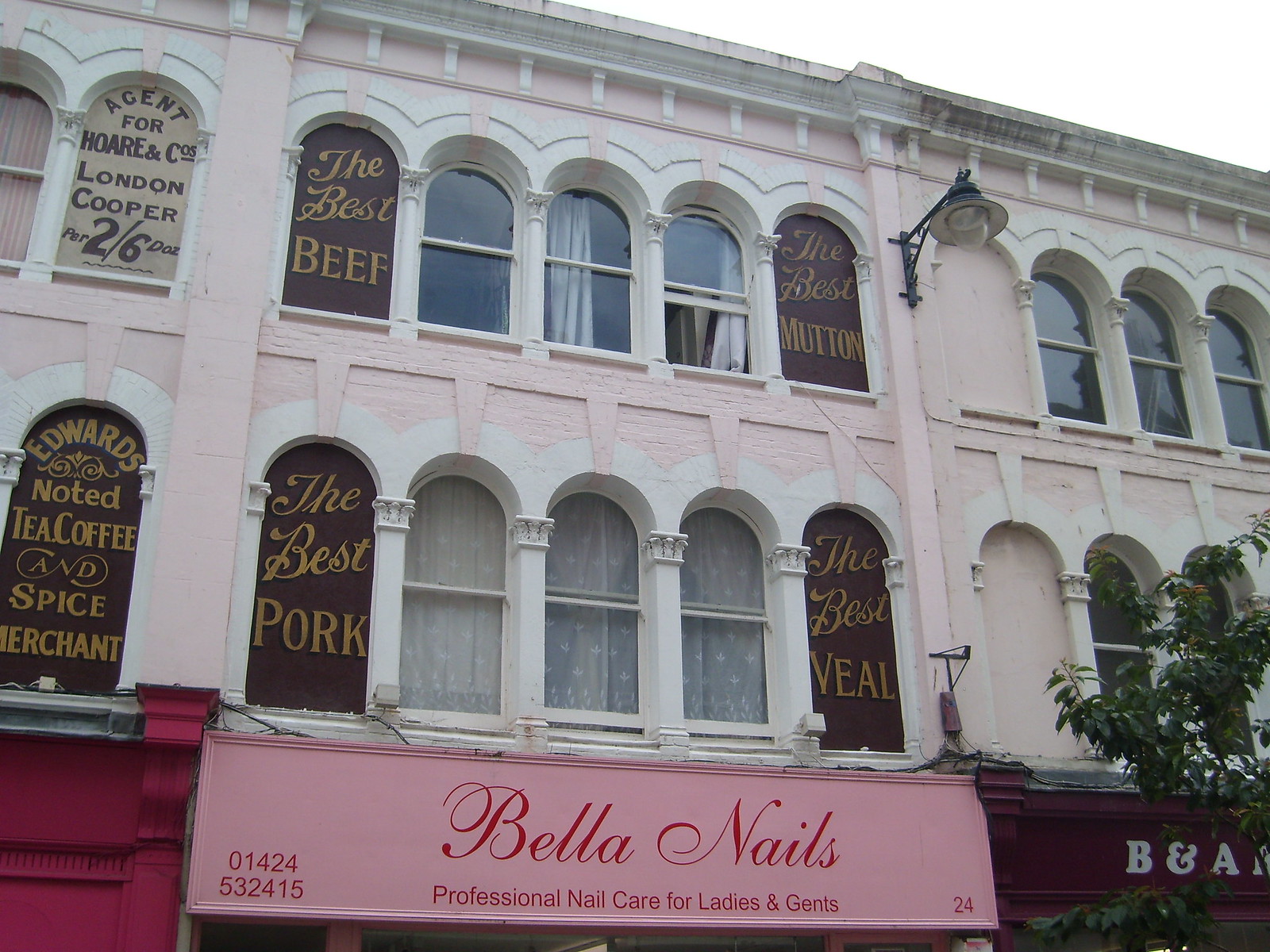The image depicts a large multi-story building, constructed primarily of brick and painted in a light, pretty pink color with white trim. The architecture features beautiful windows with arched tops, adorned with vintage or historical-looking lettering. Several windows display historical advertisements: "The best beef, the best mutton, the best pork, the best veal," while others announce, "Agent for Horne and Companies, London Cooper" and "Edwards Noted Tea, Coffee, and Spice Merchant." These signs are stylized in brown and gold, giving a nod to early 20th-century design.

On the ground floor, beneath an awning, is a vibrant beauty parlor marked by a hot pink sign that reads, "Bella Nails, Professional Nail Care for Ladies and Gents," written in fancy script. This establishment captures a charming mix of historical elegance and modern business.